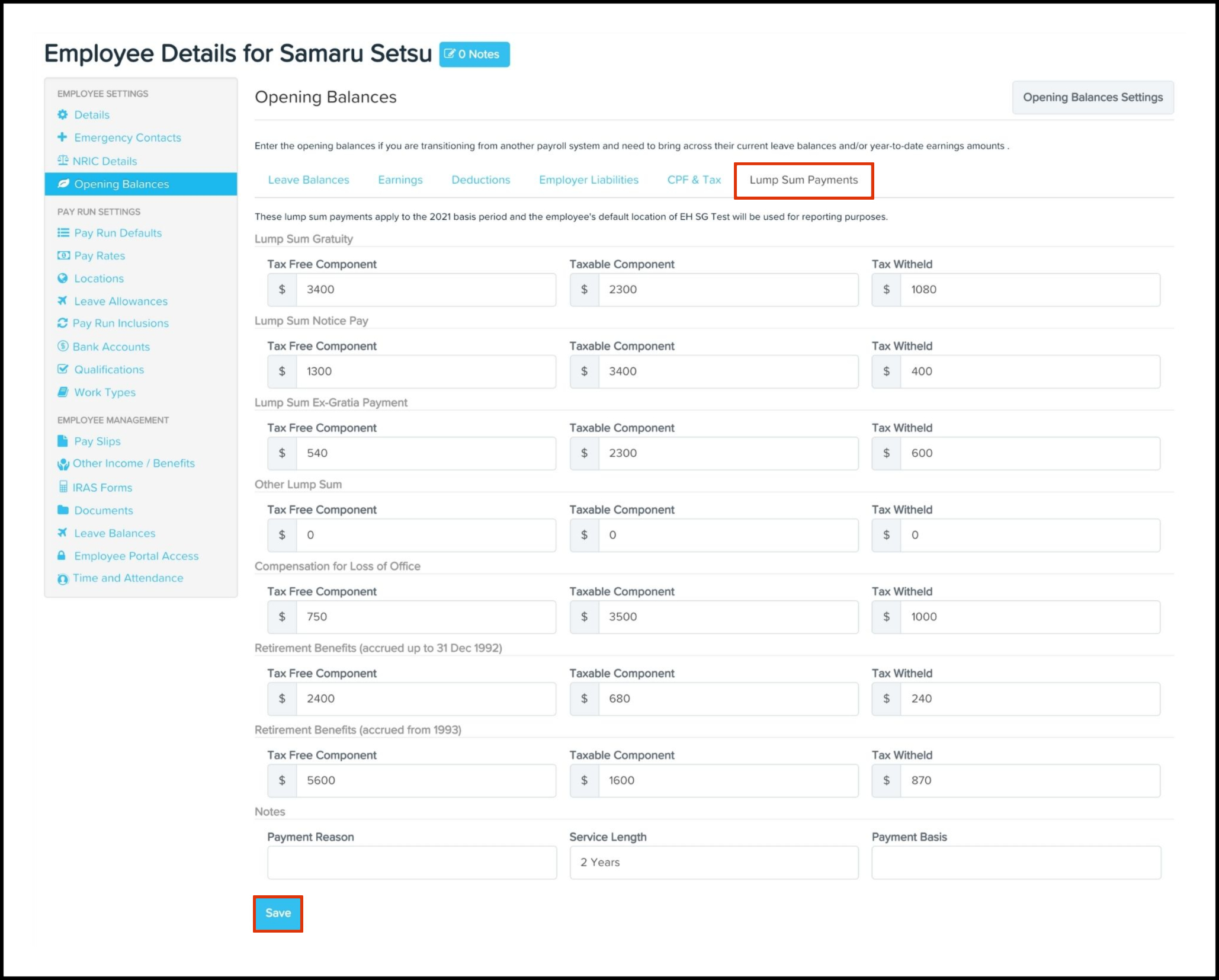### Detailed Caption for Image

The image showcases a computer screen displaying employee details for "Samaru Setsu." It presents a detailed breakdown of various financial components, particularly focusing on opening balances, which are essential for transitioning from another payroll system and maintaining accurate leave balances and year-to-date earnings.

Prominently highlighted in bold letters are sections labeled "Leave Balances," "Earnings," "Deductions," "Employee Liabilities," "CFF and Tax," and "Lump Sum Payments." Notably, the information on lump sum payments is provided with specific details for the 2021 basis period, and reporting utilizes the default employee location "EHSG Test."

Several financial categories are elaborated upon within these lump sum payments:
1. **Lump Sum Gratuity:** 
    - **Tax-Free Component:** Example amounts such as $3,400 are indicated.
    - **Taxable Component:** Example amounts such as $2,300 are indicated.
    - **Tax Withheld:** Example amounts such as $1,080 are indicated.

2. **Other Lump Sum Payments:**
    - An additional category includes a **tax-free component** of $540.
    - The **taxable component** again stands at $2,300.
    - Taxes withheld are detailed as $600.

Other categorized payments include "Lump Sum Notice Pay," "Lump Sum Ex Gratia Pay," "Compensation for Loss of Office," and "Retiree Benefits Accrued up to December 31, 1992." Each category contains specific figures, reflecting different components of lump sum payments, such as tax-free and taxable elements.

The overall document serves as a comprehensive lump sum payment report, presumably intended for printing and review.